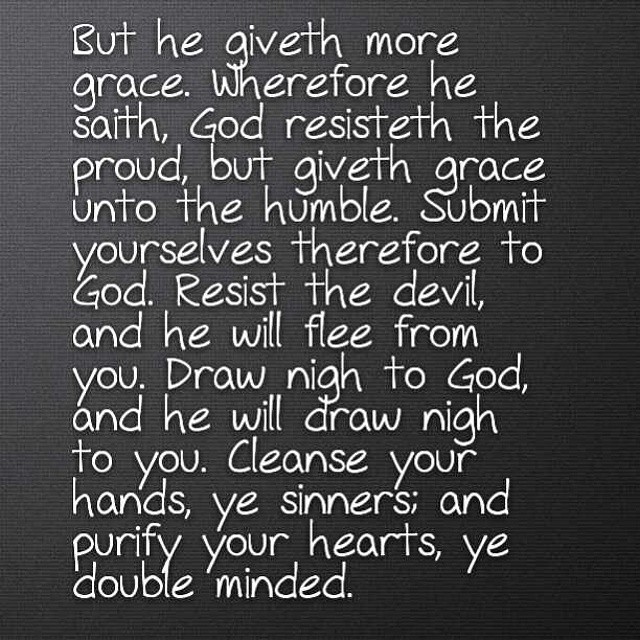This image appears to be a digitally produced inspirational card or an online post, perhaps fit for platforms like Instagram or Facebook. The background of the image transitions from dark gray to black as you move from left to right, creating a gradient effect. The text, which is the main focus, is written in white with a handwritten font. The message is a biblical passage that reads:

"But he giveth more grace. Wherefore he saith, God resisteth the proud, but giveth grace unto the humble. Submit yourselves therefore to God. Resist the devil, and he will flee from you. Draw nigh to God, and he will draw nigh to you. Cleanse your hands, ye sinners; and purify your hearts, ye double-minded."